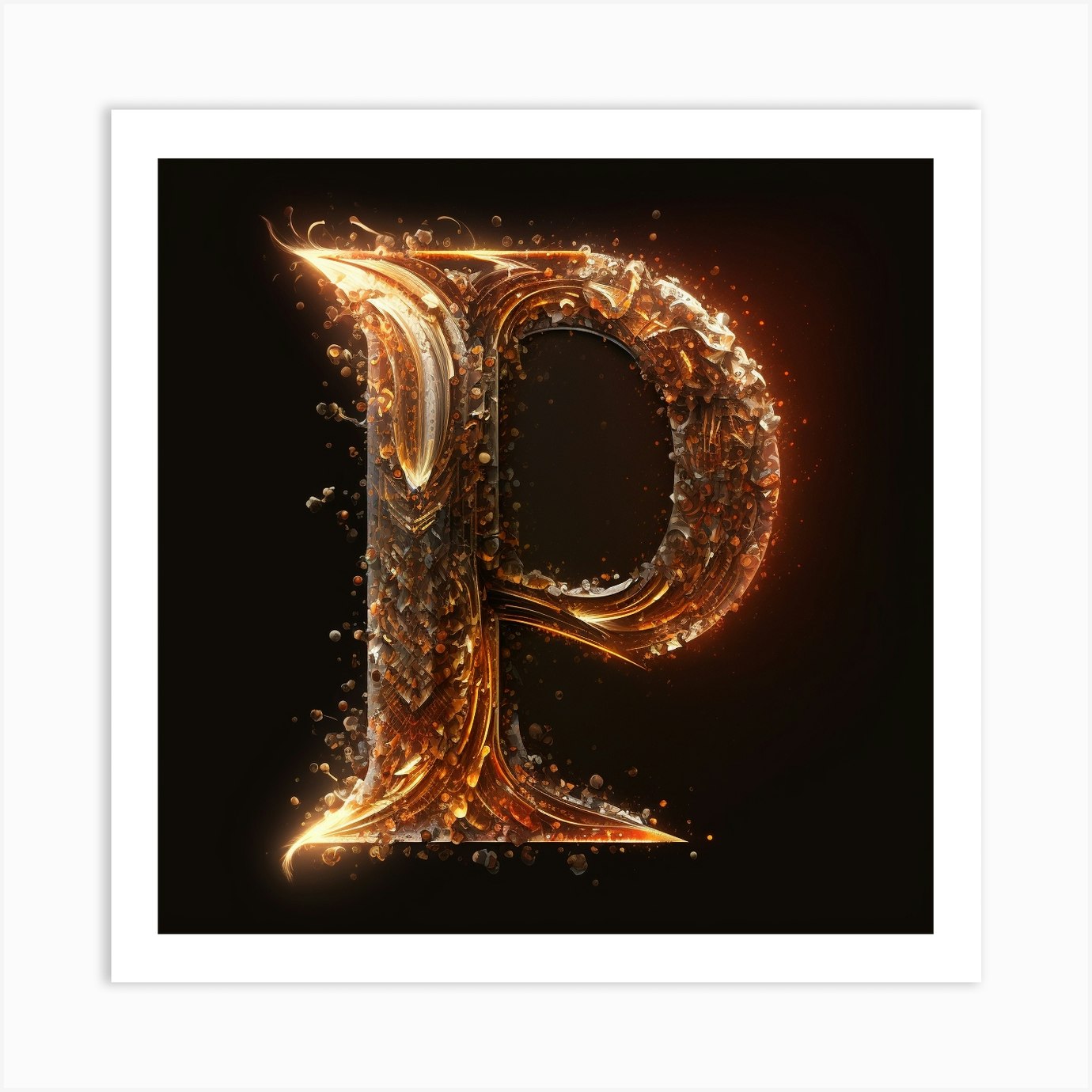The image depicts a highly stylized, computer-generated rendition of the capital letter "P" set against a black background enclosed within a white border, mimicking the appearance of a Polaroid picture. The letter "P" is large and elaborate, crafted to resemble a metallic and flaming gold texture, as if formed from molten gold. The design features gold lettering with intricate swirls and has a serif-like quality, observable at the edges where the lines flare out and form pointed tips. These points, particularly at the base and top left of the "P," give it an ornate, script-like appearance. The metallic letter also exhibits a glowing red-yellowish hue, adding to its heated, almost otherworldly effect, with small circular flecks of red and yellow that suggest flaking metal or embers. Some sections of the "P" appear to twist and turn in a serpentine manner, enhancing its fiery, dynamic essence.